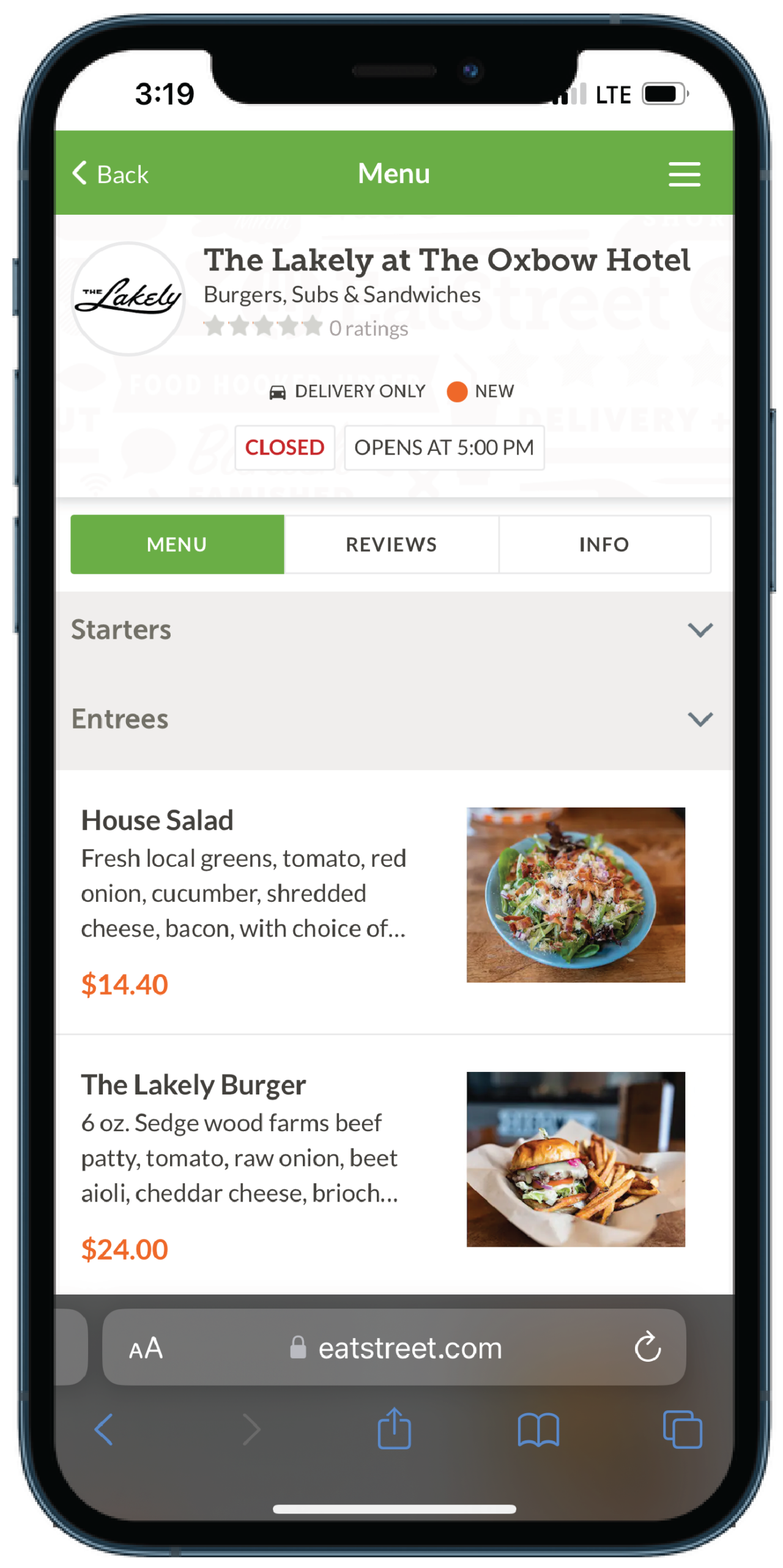In this image, we see a smartphone displaying the menu page for "Lately at the Oxbow Hotel," a restaurant chain specializing in burgers, subs, and sandwiches. The screen begins with the menu banner at the top, which features a drop-down list and a back button for navigation. Beneath the banner, the hotel’s logo is prominently displayed, accompanied by text indicating that the restaurant is new, delivery-only, and currently has zero ratings. The status shows that the restaurant is currently closed and will open at 5 p.m.

Below this section, there are three interactive buttons labeled "Menu," "Reviews," and "Info." The "Menu" section is selected, revealing subcategories including "Starters" and "Entrees." Under the "Entrees" category, two items are listed: the "House Salad," priced at $14.40, followed by the "Lately Burger," which is priced at $24. Each item features an image of the dish to the right and a brief description of the ingredients situated between the title and the price. The images provide a visual allure, enhancing the appeal of the dishes on offer.